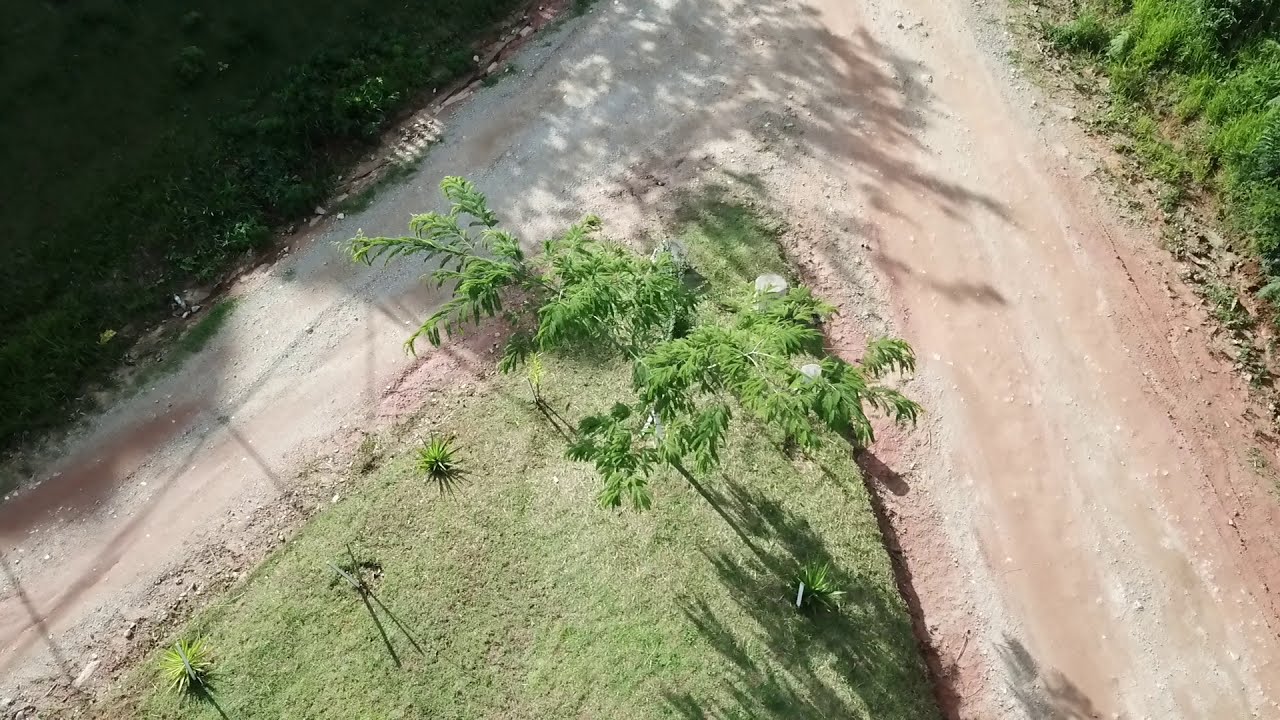This aerial photograph, taken by a drone, captures the intersection of a dirt and gravel road that forks sharply into a V-shape. The path, characterized by its reddish-pink dirt and light gray gravel, curves steeply from the bottom right of the image, meeting at a point at the top middle before diverging again towards the bottom left. Nestled within the crook of this V-shaped fork lies a triangular front yard, covered in green grass and crowned by a single small tree at its pointed tip. The perimeter of this grassy area features spiky plants resembling sea urchins, while the immediate surroundings outside the fork are filled with a diverse array of vegetation, including foot-tall broad-leaved plants and wild grasses, adding a vibrant tapestry of green and yellow hues to the landscape.